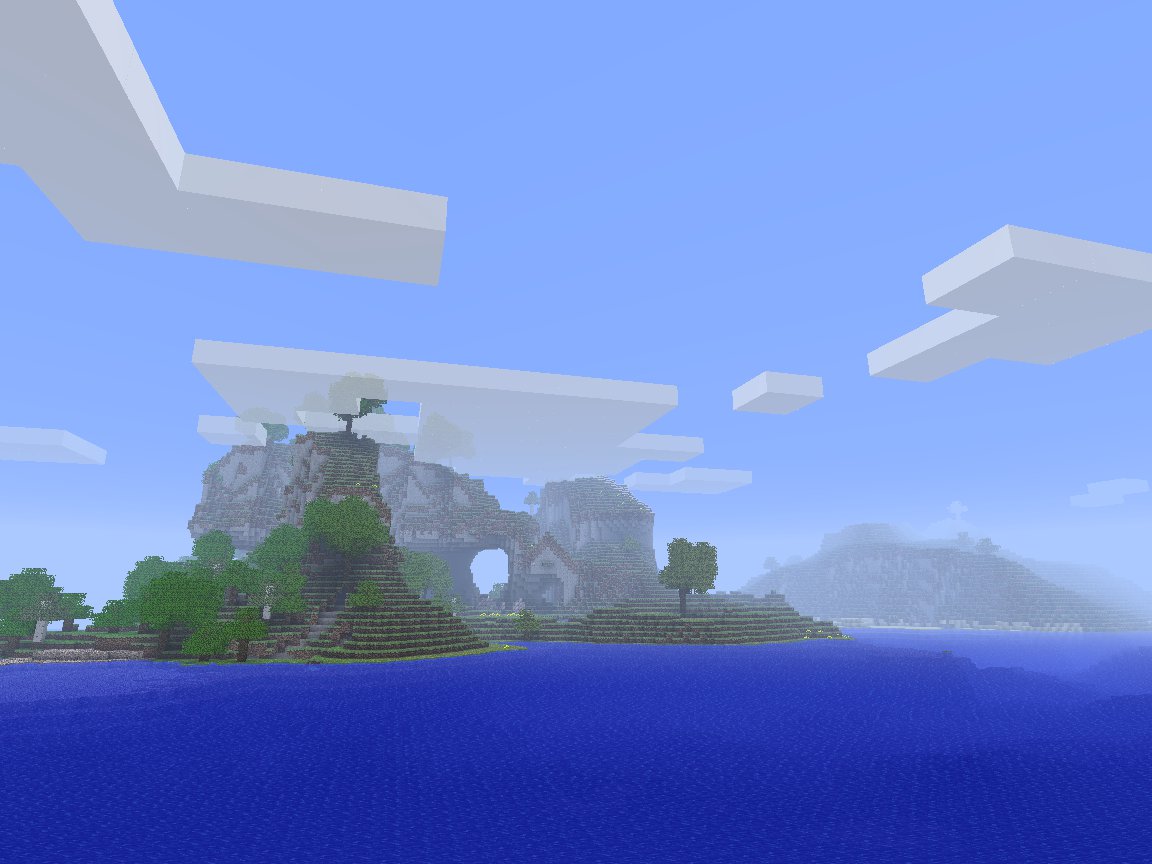A surreal, digitally-created image depicts a fantastical scene under a vivid blue sky. The clouds, composed of various solid, geometric boxes, float impossibly in the atmosphere, their sharp edges and visible sides deviating strikingly from the fluffy, natural formations we're used to. 

Below, an island of sheer rock formations juts dramatically out of a vividly blue body of water. The rock island features towering cliffs, through which one can glimpse the sky, giving the illusion of transparency. Atop the island, a structure resembling an A-frame house is discernible, though its details remain ambiguous. Multiple levels of winding stairs ascend the rocky cliffs, leading up to a canopy of trees that stretch through the boxy clouds.

In the distance, more islands can be seen, heightening the image's dreamlike quality. The overall effect is a striking and fantastical portrayal of an otherworldly landscape, its surreal elements creating a captivating, yet unrealistic, visual experience.